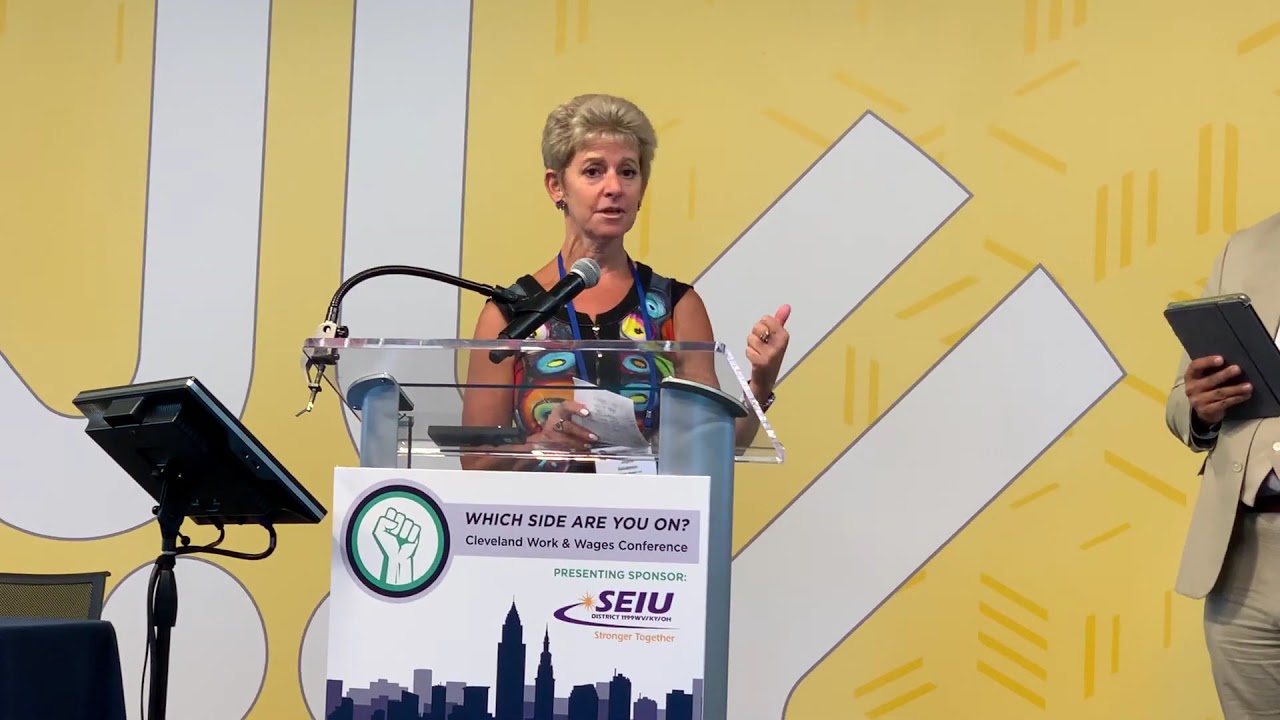In this image, a woman is center stage giving a speech at a conference. She stands at a podium that has a glass surface and displays a banner with a skyline and a fist in a blue circle, reading "Which side are you on? Cleveland Work and Wages Conference, presenting sponsor SEIU stronger together." The background is dominated by a yellow and white pattern or design that takes up the entire backdrop. The woman, who has short blonde hair and peach skin, is wearing a sleeveless dress with a vibrant mix of colors—black, green, light blue, orange, yellow, and touches of red. She holds notes in her right hand, and her fingernails are painted white. Mounted on the podium in front of her is a black microphone and a teleprompter. Just to the right side of the image, you can see the partial figure of another person dressed in a tan suit and holding a black iPad, with only the right half of their body visible up to their shoulder and down to their knee.